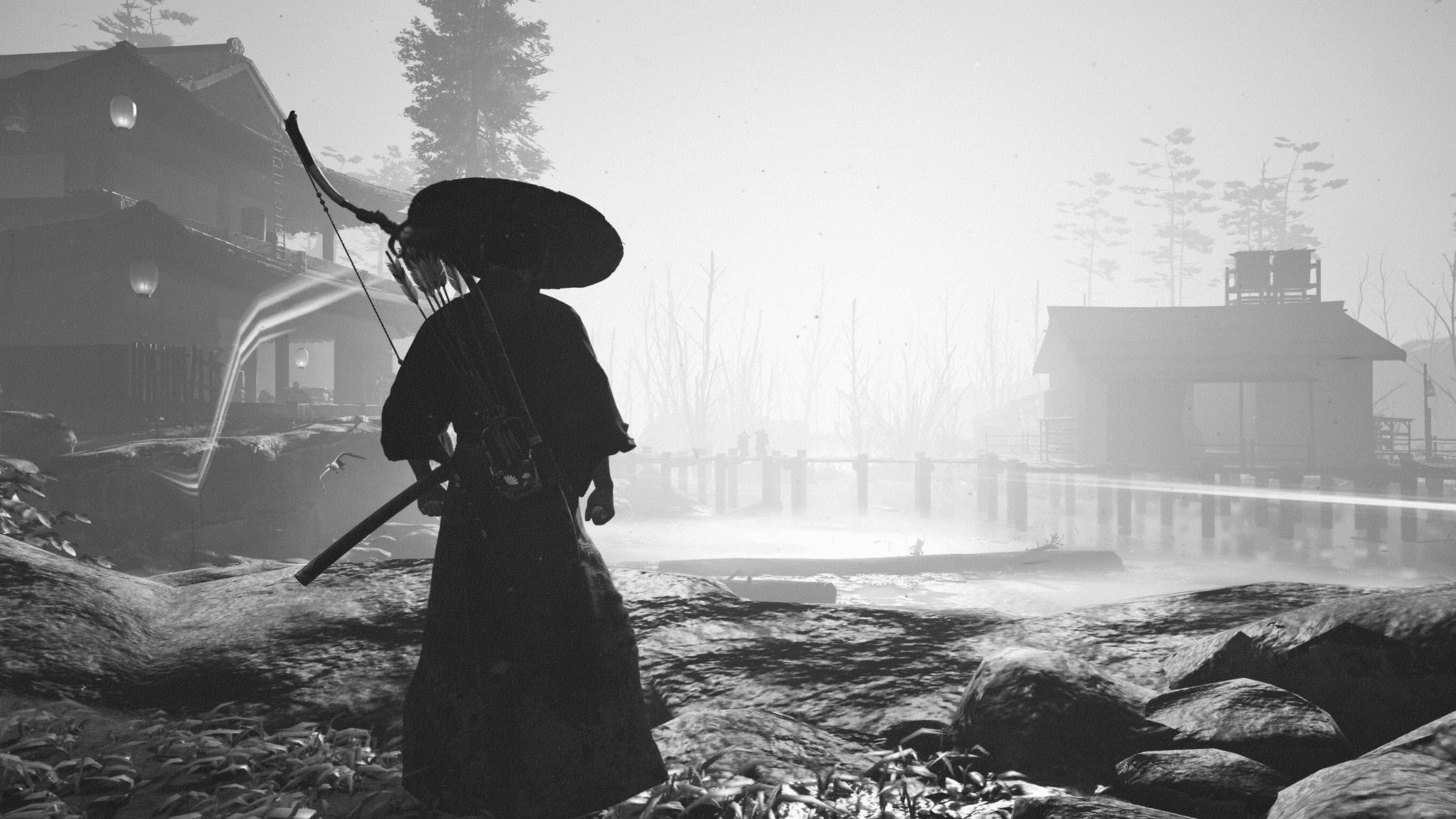A hauntingly evocative scene, this black-and-white photograph captures a solitary figure standing amidst a dreamy, almost surreal landscape. The person, who might be a woman, is cloaked in deep shadows, rendering their features and attire indistinguishable except for the vague outline of what seems to be a frilled dress and a large, round hat. They stand turned, gazing into the distance, enveloped in a thick, hazy atmosphere that blurs the boundaries between reality and fantasy.

Framed perfectly, the figure is positioned at the forefront, drawing the viewer's eye immediately to their enigmatic form. In the background, a quaint fence runs horizontally, guiding the eye towards a modest house that settles into the backdrop, almost ghostly in its undefinitive shape. On either side of the house, two trees stretch upwards, their branches fading into the haze. To the far left of the image, a larger structure looms mysteriously, its details lost in the mist, adding an element of intrigue and perhaps even foreboding.

The entire composition, drenched in grayscale tones, exudes a cinematic quality reminiscent of classic films. The contrasting elements—the clear outline of the figure and the nebulous background—create a mood of introspection and mystery, sparking curiosity about the story behind this captivating image.